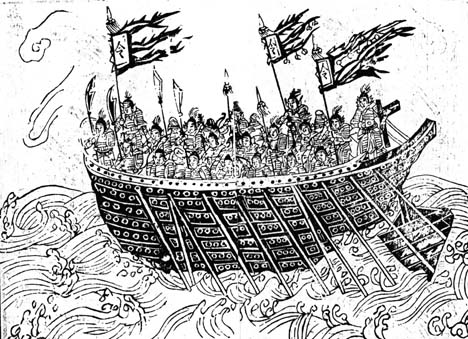The image is a black-and-white hand-drawn or possibly hand-blocked illustration of an old-style warship, centered in a choppy, stormy sea with violent waves. The boat, intricately carved and densely packed with adult soldiers, stands out in the middle of the frame. Blowing in the wind are three flags with rectangular shapes and tassels or dragon tails. The soldiers, likely of Asian origin, are armed with various weapons, including spears, large poles, swords, and other sharp-edged implements. Numerous oars extend from the boat, indicating manual rowing, and a person is seen steering at the back, emphasizing the traditional and historical essence of the scene. The sky is mostly white with a few clouds in the top left corner, enhancing the dramatic atmosphere of this detailed and possibly Asian-inspired artwork.